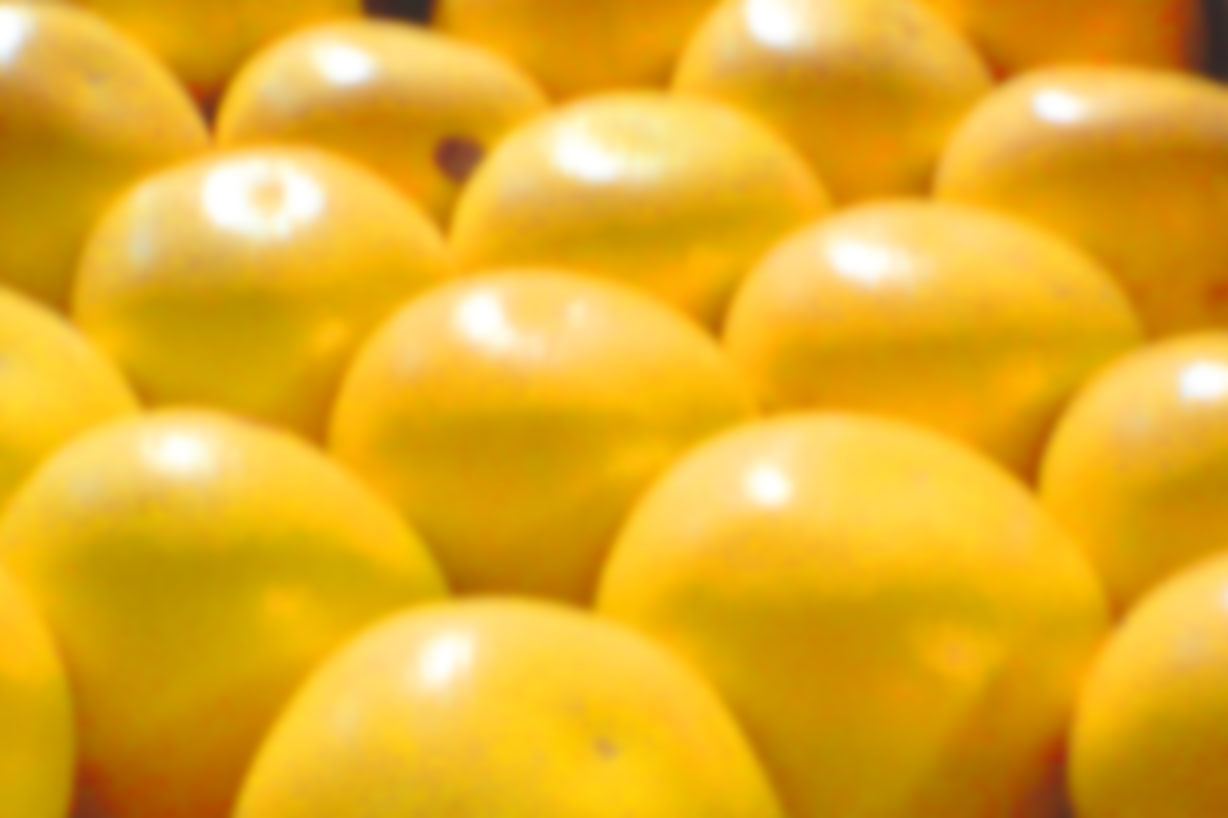The image displays a close-up of approximately 18 yellow, sphere-shaped fruits, potentially lemons, tangerines, or tangelos, tightly packed together. The fruits are illuminated from above by a bright light, reflecting off the tops of the spheres and casting pronounced highlights. Some fruits exhibit black or dark spots and small dimples at their peaks. The photo appears to be somewhat blurry and reveals a dark shadow in the top right corner, suggesting possible light sources like a round lamp or a heat lamp above the scene.